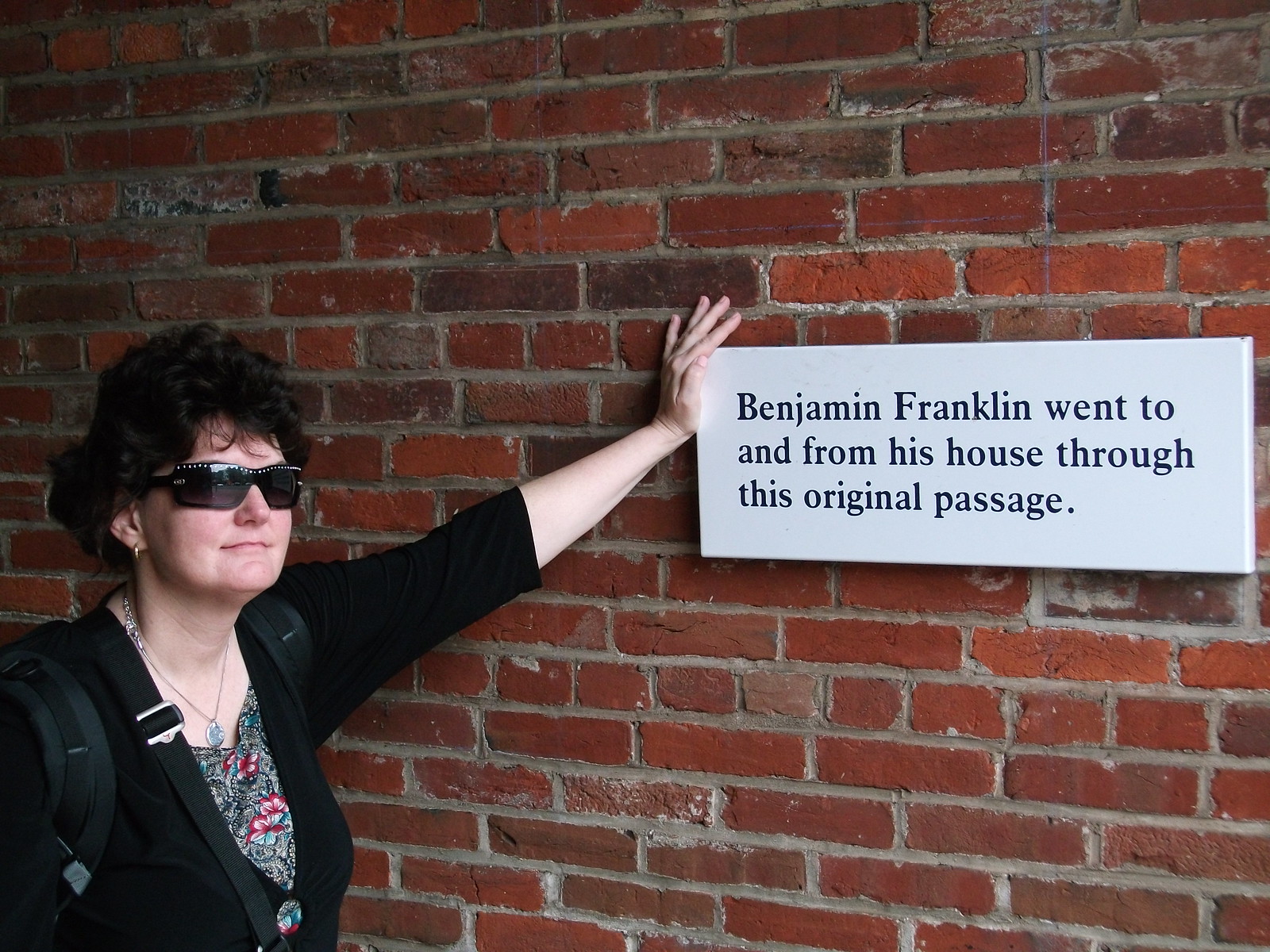In this daytime photograph taken outdoors, an old red brick wall with graying grout forms the backdrop. The wall, displaying various shades of red, is illuminated from the right-hand side, creating a gradient of light across the bricks. Centered in the image is a white rectangular informational plaque with black text, reading: "Benjamin Franklin went to and from his house through this original passage." 

Standing to the left of the plaque, a woman of Caucasian descent is featured. She has short, curly black hair and wears black sunglasses, a black sweater over a floral print blouse, and a black backpack, visible by its straps. Her right hand is gracefully extended, touching the corner of the plaque with her thumb. She gazes directly ahead, possibly at the person taking the photograph.